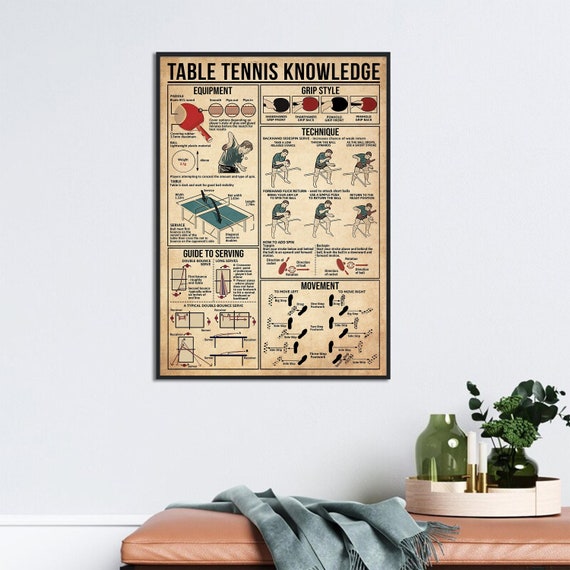A digitally edited product photo showcases a detailed, retro-style poster diagram filled with comprehensive table tennis knowledge. The off-white, aged-looking paper, featured within a black frame on a white wall, outlines intricate breakdowns of equipment, grip styles, techniques, serving guides, and movement methods. Each section includes precise illustrations, such as a red and black paddle, green table, different hand grips, serving methods, human figures demonstrating techniques, and movement footprints. Positioned in what looks like an entryway hallway, the scene below the frame includes a brown leather bench with a gray-blue scarf and two vases, one empty and one with green plants, enhancing the decor.